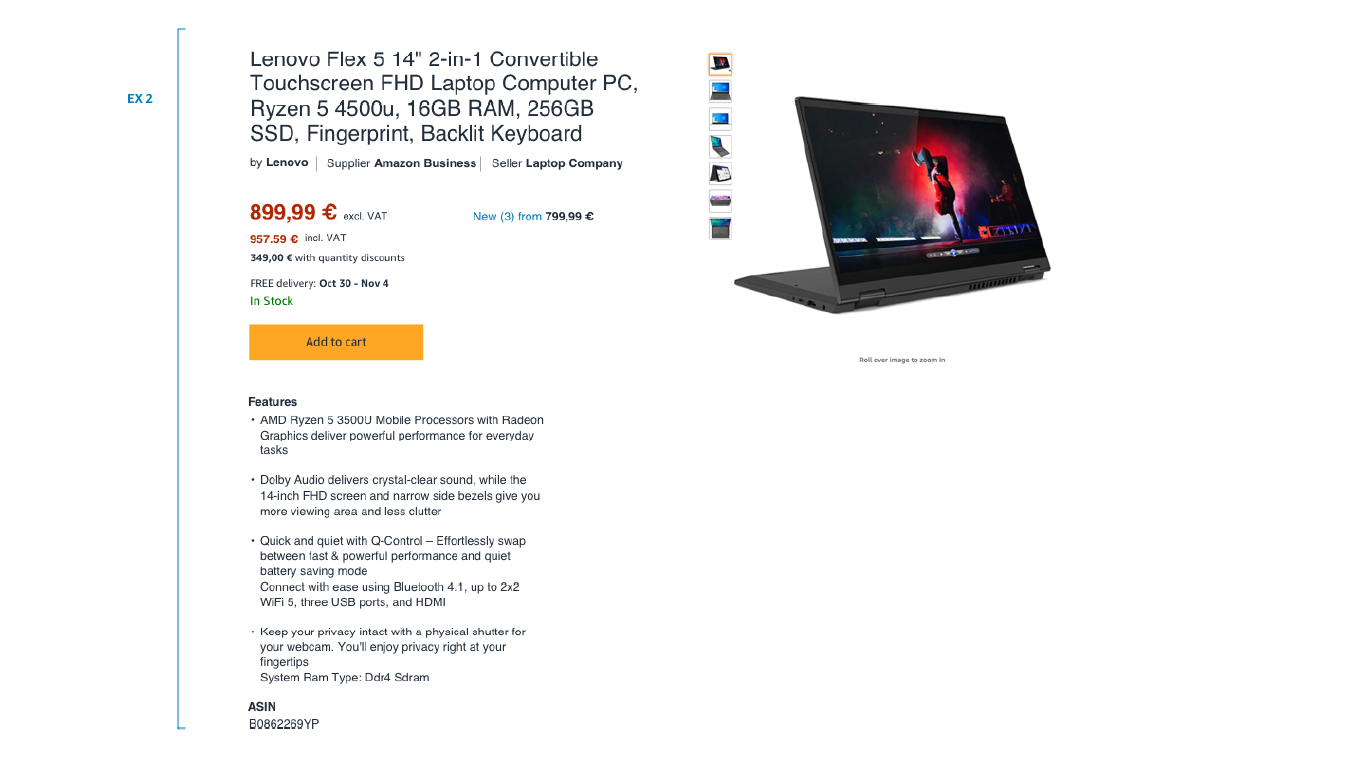A detailed listing image is displayed on a laptop screen for a Lenovo Flex 5, 14-inch 2-in-1 convertible touchscreen FHD laptop. The webpage's layout and color scheme are reminiscent of Amazon's style, though only the specific product details can be clearly ascertained. On the right-hand side of the screen, there's an image of the gray-colored Lenovo Flex 5 showcasing a vibrant red and black graphic on its display. To the left, detailed specifications and selling information are provided.

The laptop is described as a Lenovo Flex 5, equipped with a 14-inch Full HD touchscreen, powered by an AMD Ryzen 5 4500U processor, and supported by 16GB RAM and a 256GB SSD for storage. Additional features include a fingerprint reader and a backlit keyboard. The seller is identified as Amazon Business, and the price listed is €899.99. The listing notes that free delivery is available between October 30th and November 4th, and that the item is currently in stock with an option to add it to the cart.

The product description highlights several key features: the AMD Ryzen 5 3500U mobile processors with Radeon graphics provide robust performance for everyday tasks while Dolby audio ensures crystal clear sound. The 14-inch screen with narrow side bezels offers an expansive viewing area with minimal distraction. It also mentions Lenovo's Quick and Quiet Q control, which allows users to toggle between performance and battery-saving modes. Connectivity options include Bluetooth 4.1, up to Wi-Fi 2.2, and 5 USB ports. For privacy-conscious users, a physical shutter for the webcam ensures privacy protection.